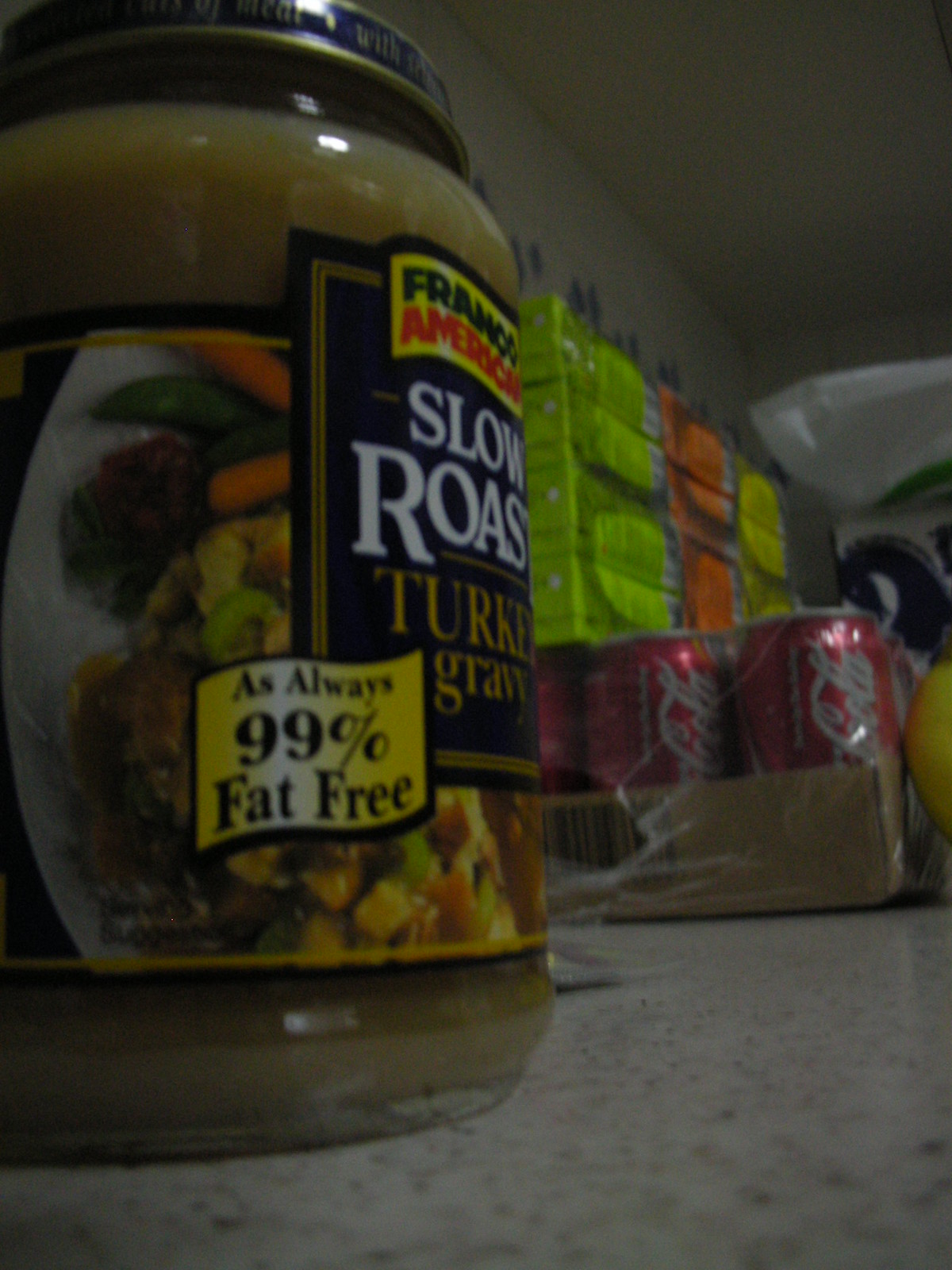In this vertically oriented rectangular image, we observe a counter laden with various food items, situated in a dimly lit room. The countertop, made of white-flecked marble, stretches across the frame. Prominently positioned in the lower front half of the image is a jar of slow-roasted Franco-American turkey gravy, showcasing its label toward the right. The close-up captures the intricate details of the jar, with its blue-capped lid reaching the top of the image. To the right of the gravy jar, a background array of stacked green, orange, and yellow boxed items adds color and depth to the scenery. Additionally, positioned in the lower right corner beneath the gravy jar, a cardboard box filled with red cans of Coca-Cola soda can be seen, hinting at an assortment of beverages and consumables present on the countertop.